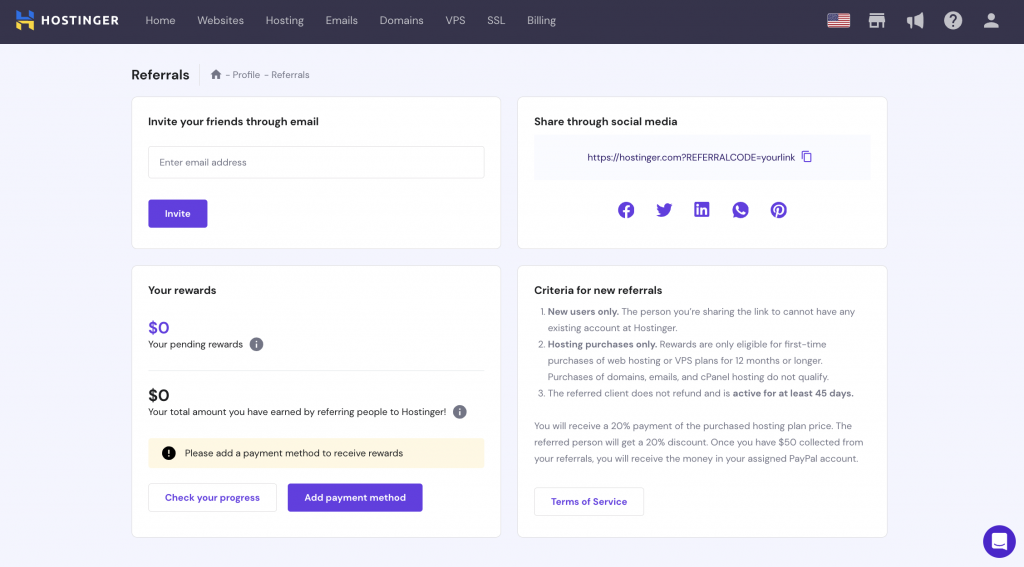This image captures the referral page of the Hostinger website, providing a detailed view of the user interface and navigation options. At the top, there are tabs labeled Home, Websites, Hosting, Emails, Domains, VPS, SSL, and Billing. On the right side of the navigation bar, icons are displayed, including an American flag, a brick-and-mortar building, a megaphone, a question mark, and a silhouette representing the login option.

The main section of the page is dedicated to the referral system and user profile. At the top, there are buttons for navigating Home, Profile, and Referrals. A prominent box allows users to invite friends via email for referrals. Below this box, users can see their rewards status, which in this instance shows $0 for both pending rewards and total earnings from referrals. It also prompts users to add a payment method to receive future rewards, with a button provided for this task.

To the right, there is an option to share the referral link on various social media platforms, including Facebook, Twitter (X), LinkedIn, Pinterest, and even via phone. Towards the bottom, there is an unreadable list of criteria for new referrals and the terms of service related to the referral program.